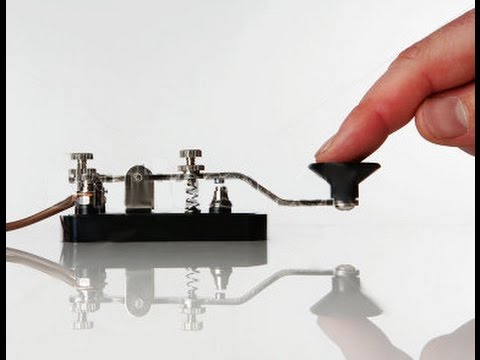The image depicts a Morse code machine placed on a flat, shiny surface that reflects both the machine and the finger of a person ready to operate it. The Morse code device, commonly known as a telegraph key, features a black base with shiny metal components, including a metal lever that culminates in a cone-like knob at the end. This knob, which the person’s finger is resting on, is used to generate Morse code by pressing it down. The machine has a clear wooden base, secured by two screws, and is connected by a brown wire. The photo includes two black borders on either side, with the person’s index finger and thumb partially visible, poised to create either a short or long press, essential for forming Morse code letters and words.